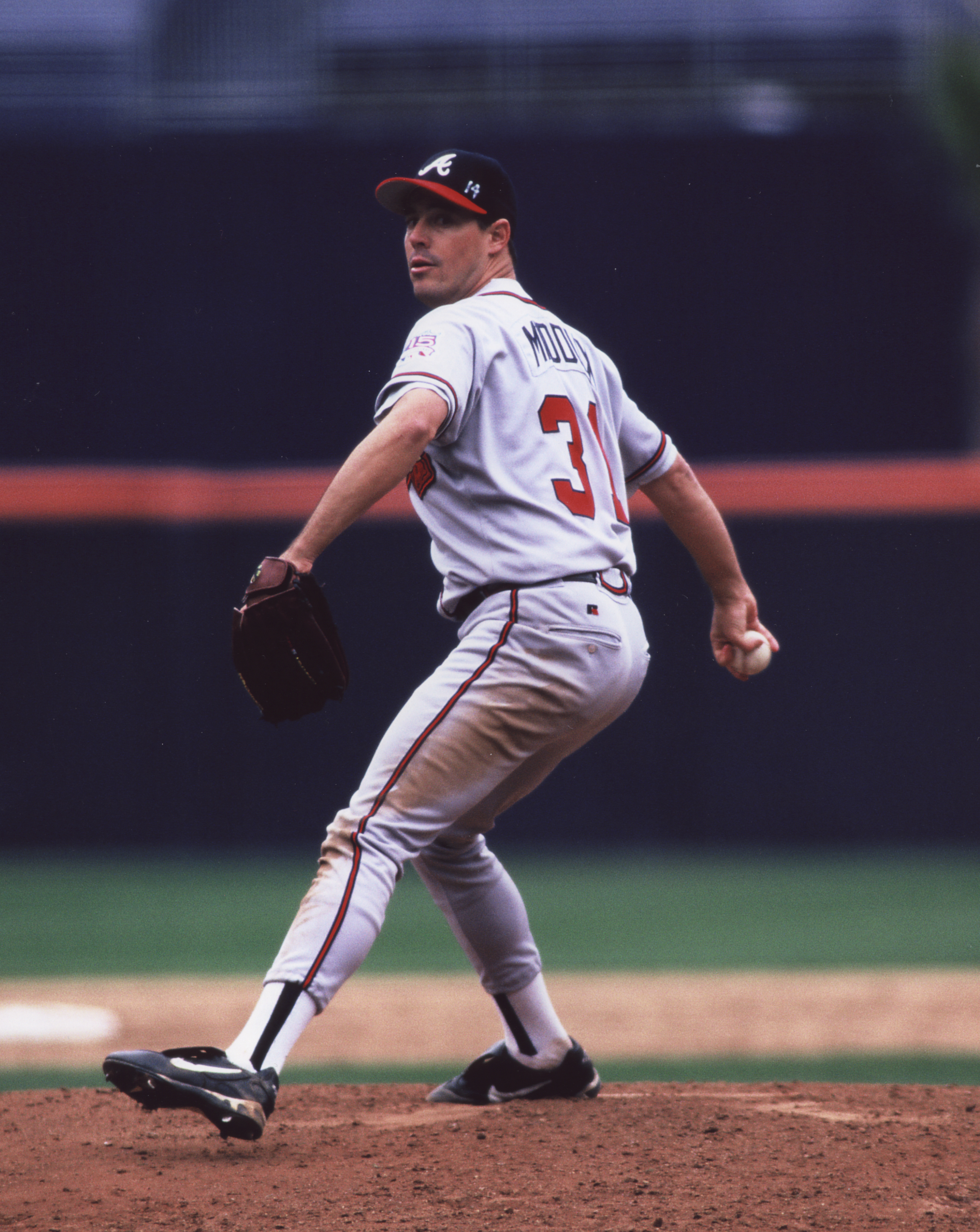The photograph captures Maddox Gregg, a baseball pitcher, poised mid-game on a dirt mound. He is preparing to throw a baseball, with his right hand gripping the ball and his left hand donning a brown glove. His body is coiled, left foot lifted off the ground, and he is focused on his target in the distance. Maddox is clad in a white jersey with red numbers, indicating the number 31 on his back, accompanied by gray pants marked with dirt stains, evidence of his efforts on the field. He wears black and white socks with cleats and a distinctive baseball cap bearing a large "A," designed in black with red accents. The background features a blurry blue and green wall, highlighting Maddox in sharp focus, emphasizing his intent and concentration.